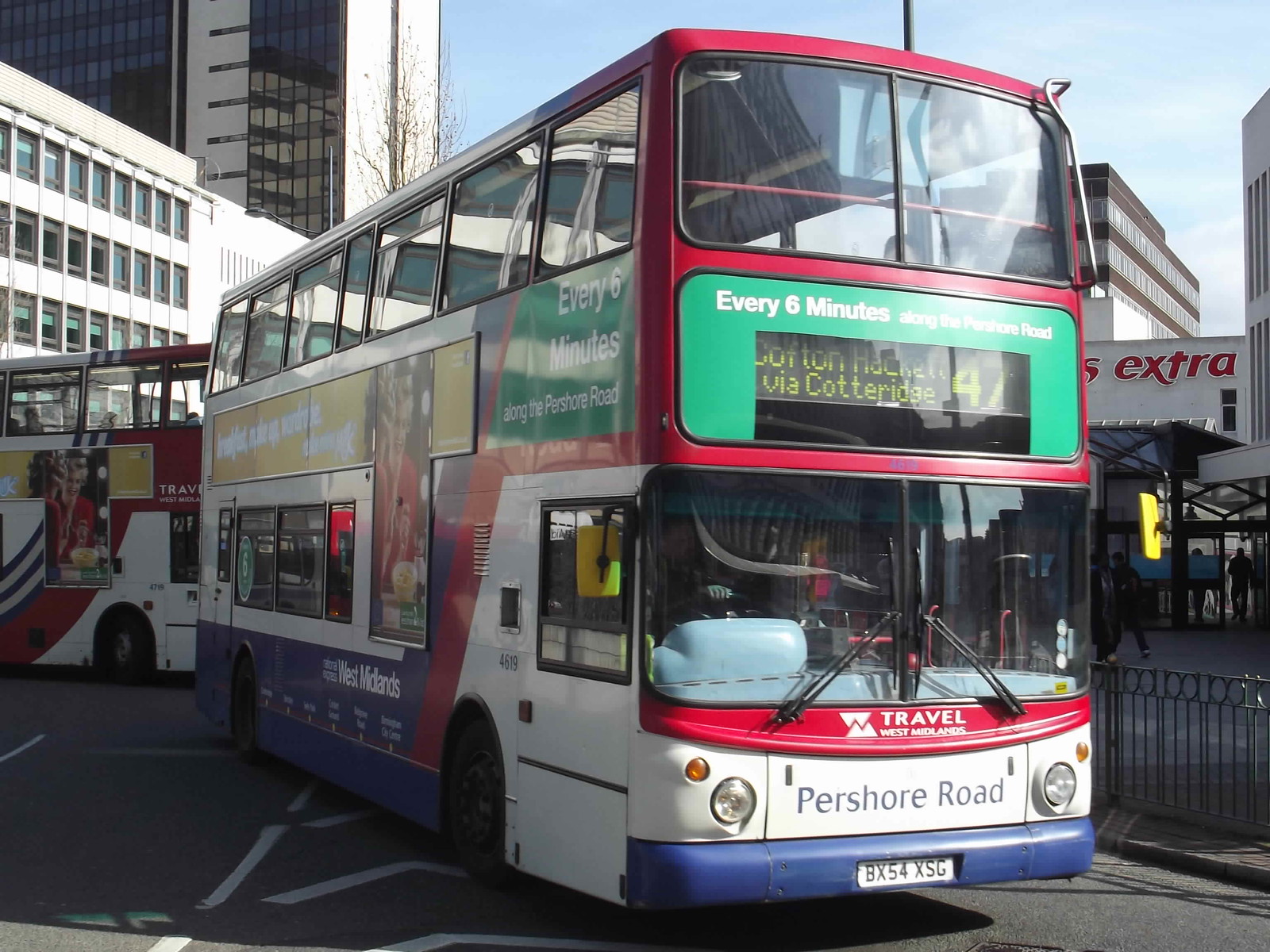The image captures an urban scene featuring two double-decker buses on a bustling city road. The primary focus is on a vividly colored bus primarily painted in red, with a green section across the middle. On this green section, a message in white reads "Every six minutes along the Pershore Road." Below this, an electronic screen displays "Coffden Hackle via Cotteridge" in yellow along with the bus number 47. The front section beneath the driver features text in white, "Travel West Midlands," and another sign in blue on a white background indicates "Pershore Road." The bus's number plate reads BX54XSG. Positioned behind is another double-decker bus, similarly adorned with red, white, and blue colors, featuring billboard advertisements on its side. 

The surroundings include a roadway filled with people walking along sidewalks lined with railings. The scene is set under a predominantly blue sky with some hazy white clouds. To the left, a towering corporate skyscraper with numerous windows reflects the cityscape. The infrastructure and the activity suggest a vibrant, busy urban environment.